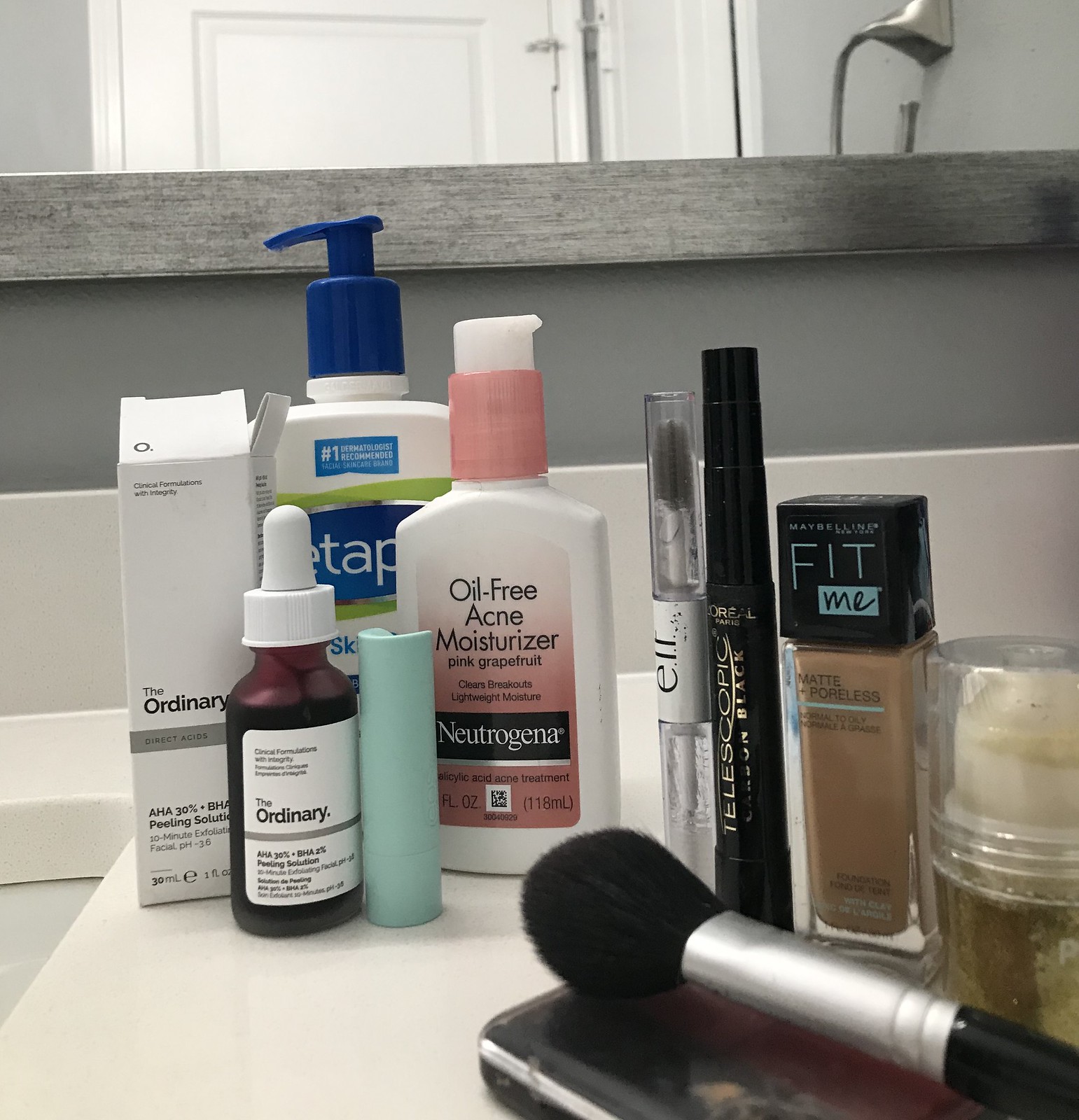This is a close-up image of a bathroom countertop. The countertop is white and features several personal care items. At the top of the picture, a mirror with a gray border is partially visible, reflecting a sliver of a white door with a silver handle. 

Starting from the left, there is an open, tall, and narrow white box labeled "The Ordinary," featuring a gray bordered section with black text. Behind the box, a lotion bottle with a blue cap, positioned to the left, is visible. The bottle has a blue label stating "number one" in white letters, surrounded by additional white text, with "Cetaphil" within a blue border in the background.

In front of the lotion bottle, there's a brown bottle with a dropper labeled "The Ordinary" with a white label and black text. To its right is a tall green cylinder, resembling chapstick.

Next, a bottle of Neutrogena oil-free acne moisturizer in pink grapefruit is present, labeled with a light pink label and a pink screw cap with a white top turned to the right. Adjacent to this are an elf makeup product and a black eyeliner, both standing upright.

Further to the right is a concealer bottle labeled "Maybelline Fit Me," featuring a black top. Beside it is a cylindrical container of glitter. Lastly, a makeup brush is laying on its side atop a case.